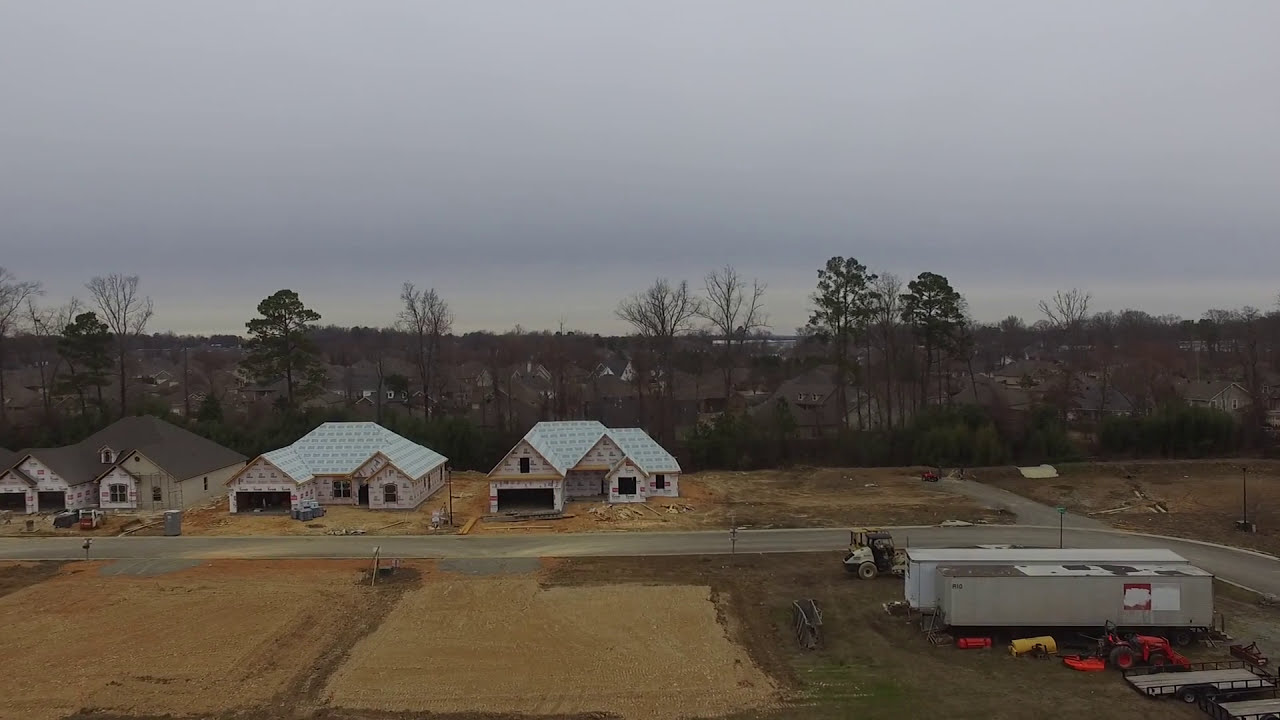This photograph captures a newly developed housing tract under construction on a cloudy, overcast day. Three two-story homes, each featuring slanted rooftops, are prominently visible from the center to the left side of the image. The houses, mostly clad in insulating material, remain unfinished without exterior siding. In the foreground, two cleared plots of land lie in front of these homes, earmarked for future development. A road winds in front of the houses and leads to the right, where several trailers, possibly used as mobile offices, and various construction vehicles, including a bulldozer and flatbed trailers, are stationed. Beyond the development site, tall trees, some barren and others still with leaves, frame the background. Through the trees, an older, established neighborhood can be seen, contrasting with the new builds in the forefront. The scene is set under a grayish-blue sky, hinting at early winter.